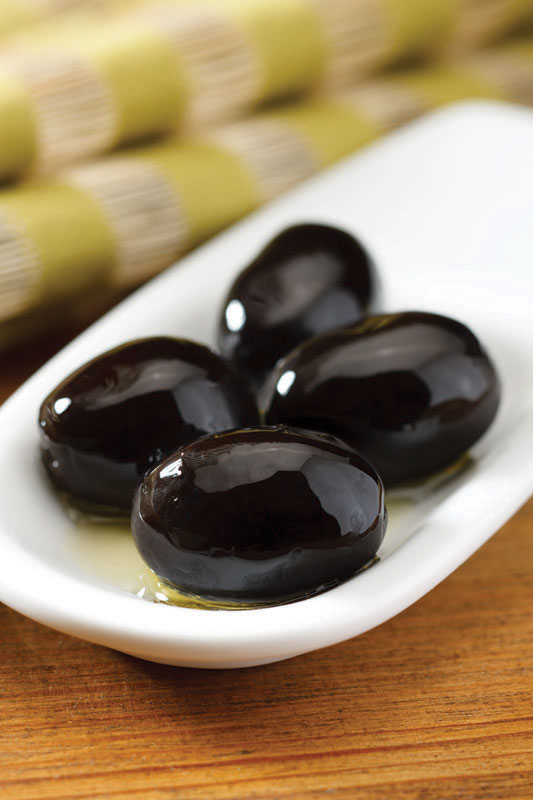The photograph showcases a small, elongated, white ceramic dish placed on a wooden table. The dish contains four black olives, arranged in two neat rows of two. The olives appear to be fresh and glistening with moisture, with olive oil pooling slightly at the bottom of the dish, giving a yellowish tint. The image is cropped closely, capturing just an inch or so of the wooden table beneath. In the blurred background, there are indistinct objects that could be rolled-up items, perhaps napkins with yellow and white rings or stripes. The image dimensions suggest it is approximately 5 inches by 3 inches.